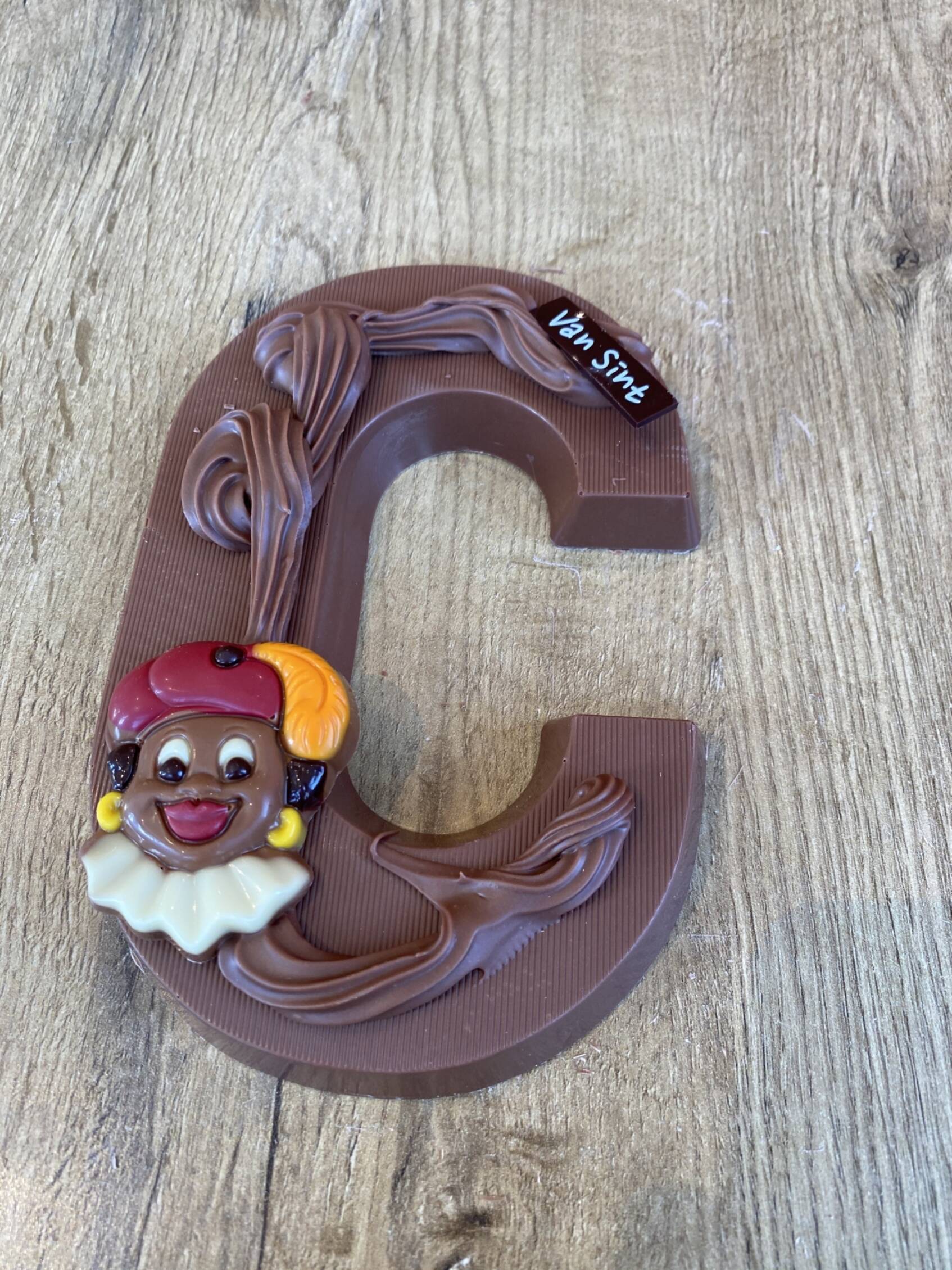A close-up image features a finely crafted piece of chocolate shaped like the letter "C," resting on a wooden table adorned with visible wood grain textures. The chocolate letter "C" is embellished with intricate swirls of frosting-like chocolate, enhancing its contoured appearance. Attached to the lower left part of the "C" is a detailed chocolate depiction of a face with distinct features: black hair, dark eyes, and red lips. The figure wears a red hat accented with an orange feather, yellow hoop earrings, and a white chocolate collar. At the top left corner of the "C," there's a small black label with white lettering that reads "Van Sint." The craftsmanship and embellishments suggest it is a meticulously decorated piece, possibly confectionery art.